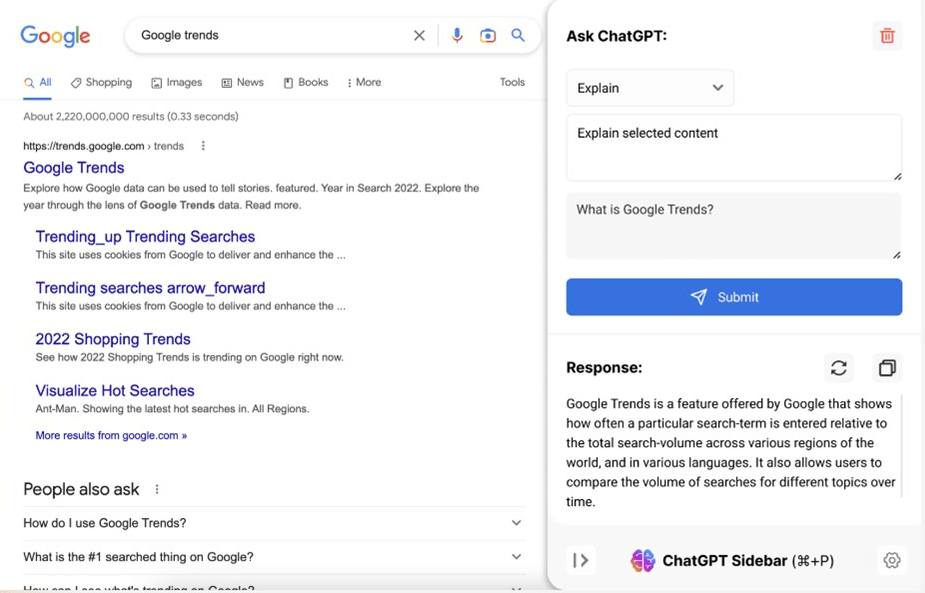A detailed screen capture of a computer monitor displaying a Google search results page dominates the left two-thirds of the image. The top left corner features the iconic multi-colored Google logo, followed by a search bar with the query "Google Trends" entered. Adjacent to the search bar on the far right are icons for voice search (a microphone), a camera for visual search, and a magnifying glass for executing the search. Directly below, a set of tabs typical in Google searches are aligned: All, Shopping, Images, News, Books, and More, with a Tools link positioned at the far right. 

The search results indicate there are approximately 2,220,000,000 results returned in 0.33 seconds. The search results are presented in bold, dark blue, almost purple text. The top result is "Google Trends," followed by links to "Trending Up Trending Searches," "Trending Searches Arrow Forward," "2022 Shopping Trends," and repeated entries for "Visualize Hot Searches." There is an additional link for more results from Google.com. 

Below the primary search results, a "People also ask" section appears, with questions such as "How do I use Google Trends?" and "What is the number one search thing on Google?"

On the far right side of the screen capture, an "Ask Chat GPT" sidebar is visible. This widget has a red trash can icon in the upper right corner. It contains three interactive fields: a drop-down box labeled "Explain," a field titled "Explain Search Content," and another asking, "What is Google Trends?" Beneath these fields is a distinctive blue button inscribed with "Submit" in white text, featuring a paper airplane icon. Below this button, the response generated by Chat GPT is displayed. At the very bottom of the sidebar, a multi-colored Chat GPT Sidebar logo is present.